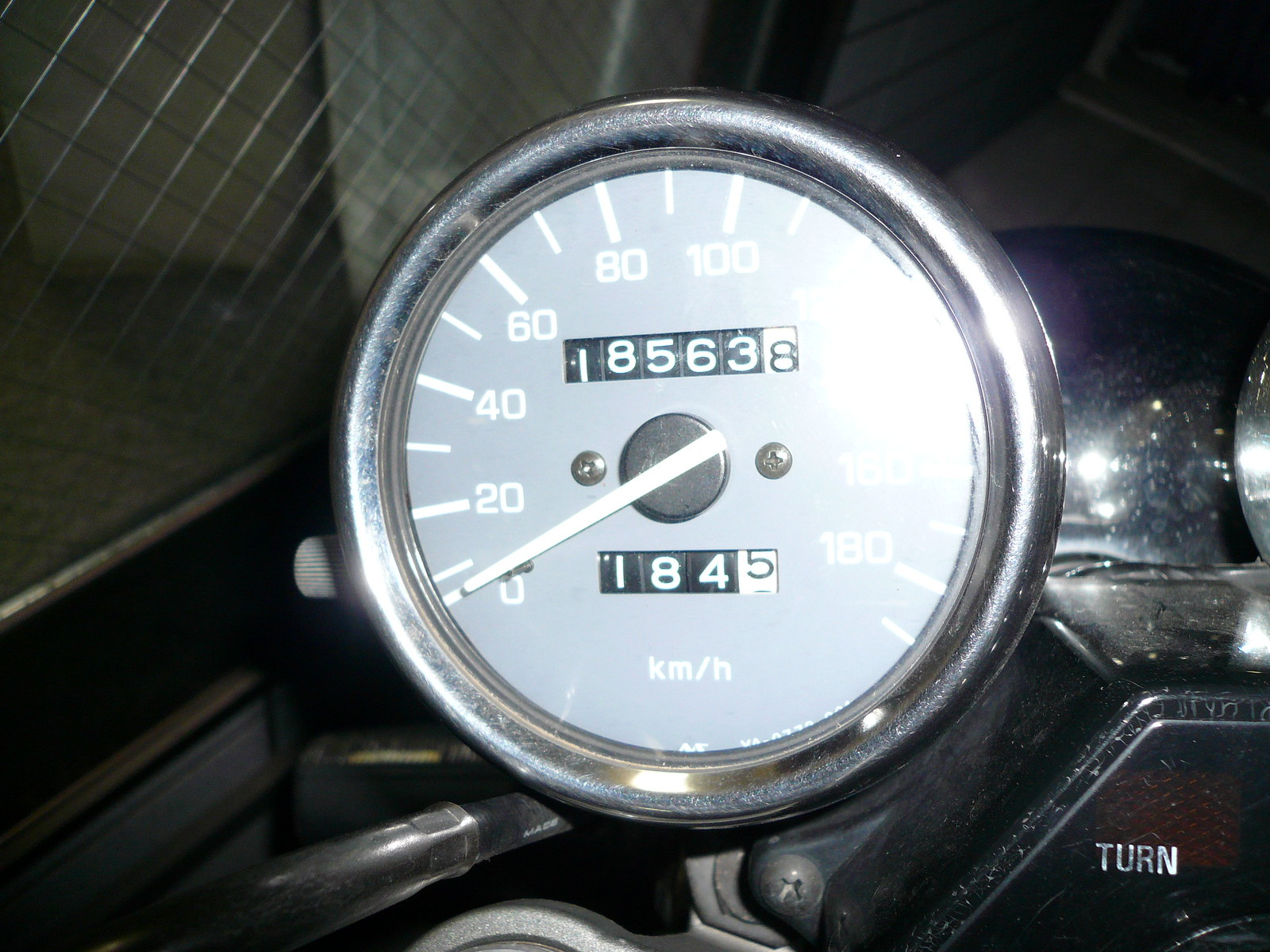The image features a close-up view of a speedometer, likely from a motorcycle or car. The speedometer displays speed in kilometers per hour (km/h) with markings at intervals of 20, ranging from 0 to 180 km/h around the circular face. The white needle, currently pointing to 0, indicates that the vehicle is stationary. The background of the speedometer is a gray-blue hue, while the numbers, dashes, and text are all in white for clear legibility. 

At the bottom of the speedometer, the text reads "km/h" to denote the units of measurement. Additionally, there are two sets of numerical readings on display: one indicating 185,638, which likely represents the total kilometers traveled, and another reading 1845, which could be indicative of a trip meter or another form of distance tracker. 

The speedometer is mounted onto a metal frame that suggests it is fixed within the dashboard or console of a vehicle, though it is zoomed-in and details are somewhat obscured. In the bottom right corner, the word "TURN" is visible, possibly referring to a turn signal indicator. Overall, the photograph captures the intricate details of a speedometer installed in a vehicle.